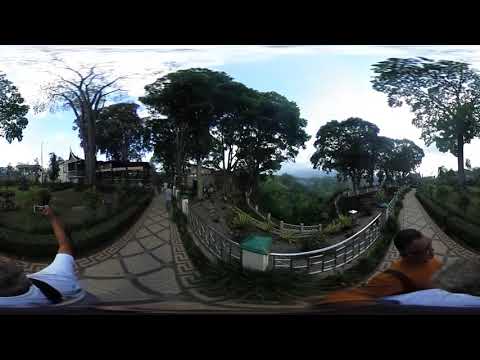The image showcases a fisheye lens perspective of a public park, possibly in an Asian country, captured in the middle of the day. A solid black border frames the picture at the top and bottom, emphasizing its 360-degree, highly warped effect. In the center of the image, a paved walkway, bordered by metal rails, stretches out, suggesting the scene is part of a bridge traversing a ravine. 

Tall trees with lush canopies surround the walkway, adding a sense of nature to the urban setting. The background reveals buildings with distinct Asian architectural elements. The sky above is partly cloudy, casting shadows that contribute to the overall darker tone of the photo.

In the lower part of the image, we see two people. One, a male, is holding a selfie stick, while the other, possibly a female, wears a light shirt and is equipped with a camera, seemingly taking a separate photograph. Scattered throughout the image are a trash can and other small objects enhancing the realism of this busy park scene. The color palette includes black, white, gray, blue, tan, and orange, adding depth and contrast to the image.